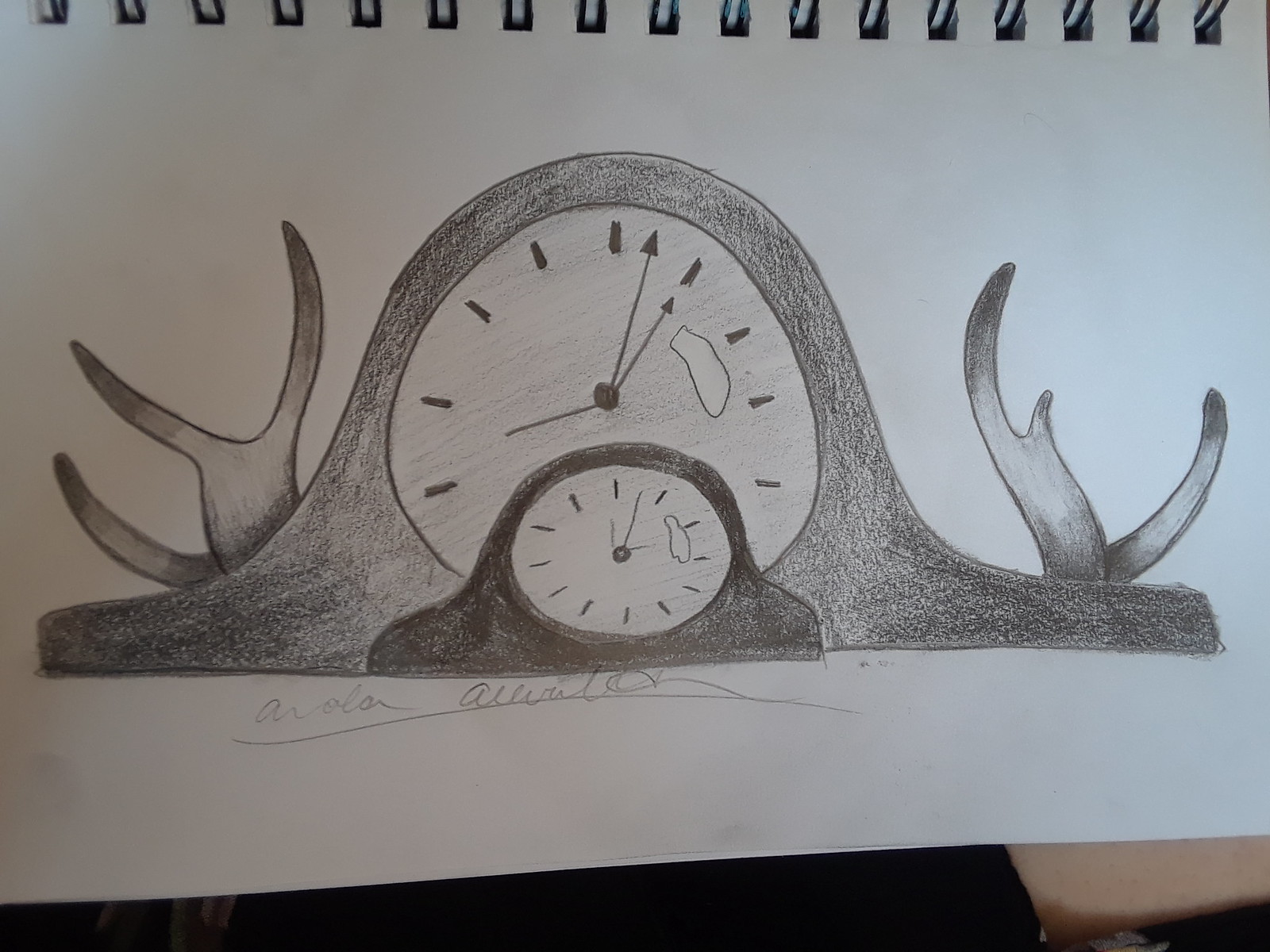This is a detailed sketch drawn on a horizontal white sketch paper with a spiral-bound top. The monochromatic drawing, executed likely with pencil or charcoal, depicts two mantle clocks reminiscent of mid-20th-century designs. The larger clock is positioned in the background, featuring a light gray face and meticulous shading to suggest depth and dimension. It shows the time as five after one and is adorned with unusual elements projecting from either side, resembling antlers or possibly stylized flames. In front of this, a smaller, darker clock reads around three o'clock, although another description suggests it might be closer to two o'clock. The drawing is signed at the bottom with a name that appears to be "Aerola" written in cursive, though it's not entirely legible. The smaller clock lacks the antler-like adornments but otherwise mirrors the design and shading details of the larger one.